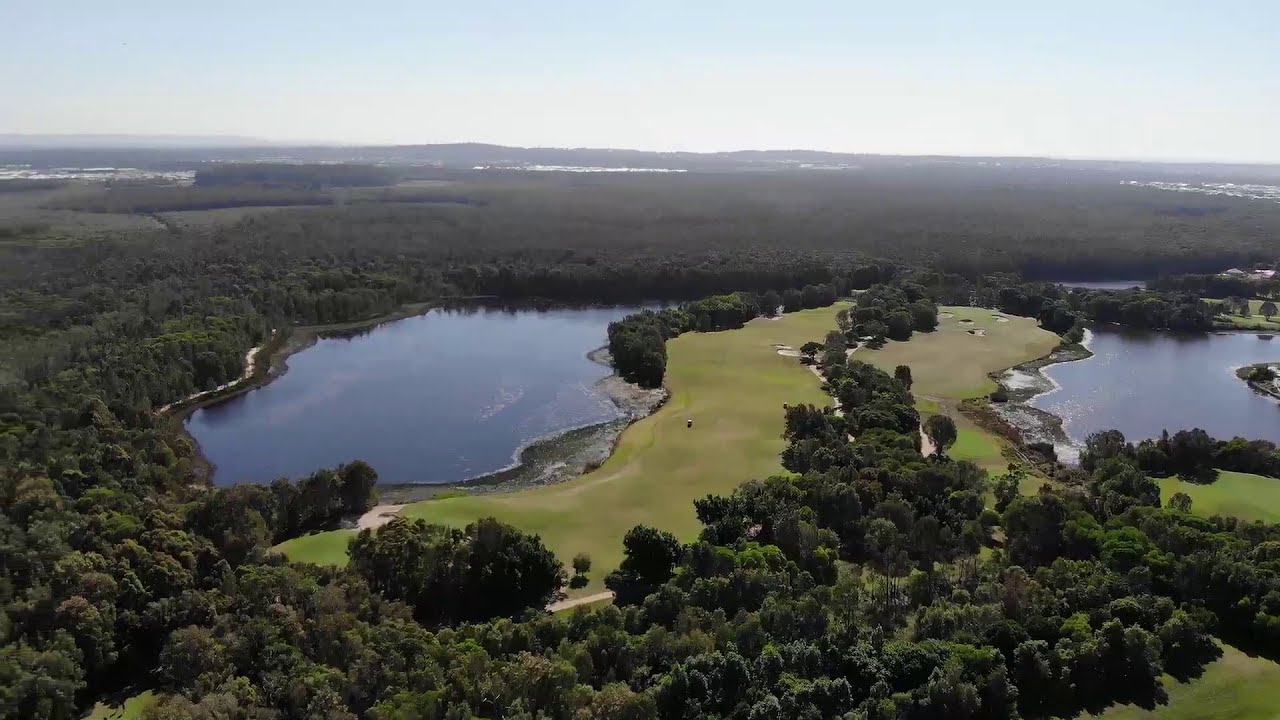An aerial photograph captures a meticulously manicured golf course nestled within a vibrant green landscape. The course is flanked by three pristine lakes, lending it a scenic and serene backdrop. The lakes encapsulate the lush fairways and sand traps, hinting at the many golf balls likely claimed by the water's edge, possibly even under the watchful eyes of local alligators. Dense clusters of large, verdant trees frame the entire scene, creating a natural border that extends outward to a seemingly endless forest, stretching all the way to the distant horizon. In the midst of the greenery, a small golf cart can be discerned, navigating the curving paths that snake through the course. Beyond the treeline, subtle hints of civilization emerge with some structures barely visible, while the horizon itself is punctuated by a distant range of mountains. Above, a clear, bright sky transitions from a soft white near the horizon to a deeper blue, capturing the brilliance of the sunlit day.